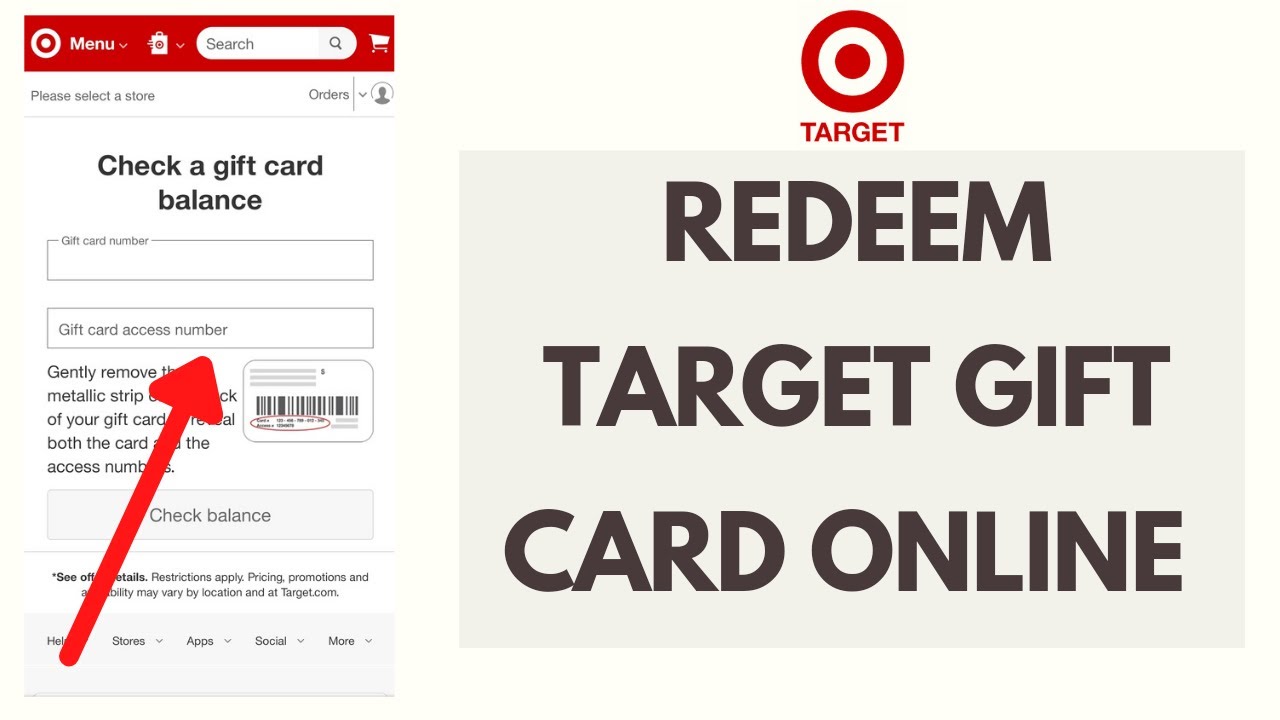In the image, there is a smartphone screen showing the Target app interface. At the top of the screen, there is a bold Target logo featuring a red circle with a red dot in the center and the word "Target" below it in red text. The background is gray, while the font is black. The text reads, "Redeem Target Gift Card Online." 

On the left side, you will see the Target menu logo button. To its right are several icons: a white battery icon, a gray search circle with the word "Search" beside it, and a white shopping cart symbol. Below this, in gray font, it reads, "Please select the store," and beside this, it says, "Orders," with a gray arrow pointing down and a gray image of a person's head and shoulders within a circle.

Further down, the text "Check a Gift Card Balance" appears, followed by "Gift Card Number" above a white square outlined in gray for inputting the details. Below this, it says "Gift Card Access Number" with a red arrow pointing to a section indicating where to gently remove the metallic strip on your gift card to reveal the card and access number.

On the right is an image showing the back of the gift card with a barcode. Beneath this, there is a gray button that says "Check Balance." At the bottom, in very small font, it reads "See offer details, restrictions apply. Pricing, promotions, and availability may vary by location and at target.com."

Finally, at the bottom of the screen, there is a gray background box with the labels "Home," "Stores," "Apps," "Social," and "More." Each label has a small gray arrow pointing down beside it.